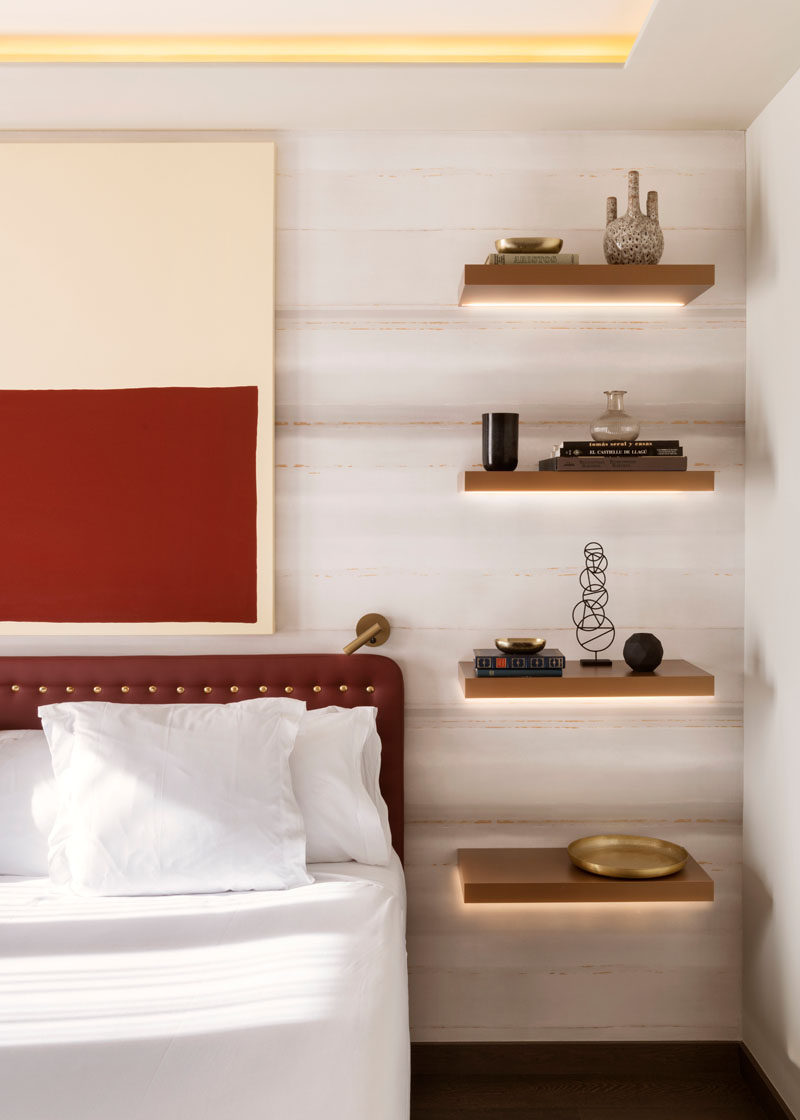This photograph, taken indoors, showcases a meticulously arranged bedroom corner with a hotel-like ambiance, highlighted by its super clean and sterile appearance. The walls are painted in horizontal stripes of muted beige and cream tones, resembling a subtle woody texture. A bed with pristine white sheets and pillows is positioned on the left-hand side. The bed features a tufted headboard in a burgundy or brick red color, adorned with shiny gold hobnails.

Above the bed hangs an abstract canvas art piece, comprised of a cream-colored rectangle with a brick red square on the bottom right. To the right of the bed, four free-floating, brown shelves protrude directly from the wall, each underlit by a light strip creating a glowing effect. These shelves are adorned with an array of decorative objects: a platinum-gold plate on the bottom shelf, books lying flat, vases (some empty), pottery, smaller baubles, and a matching gold decorative ball.

Adding to the aesthetic, a small bronze light fixture is mounted above the bed. The overall style of the room is one of photographic representational realism, meticulously staged as if for a photo shoot.